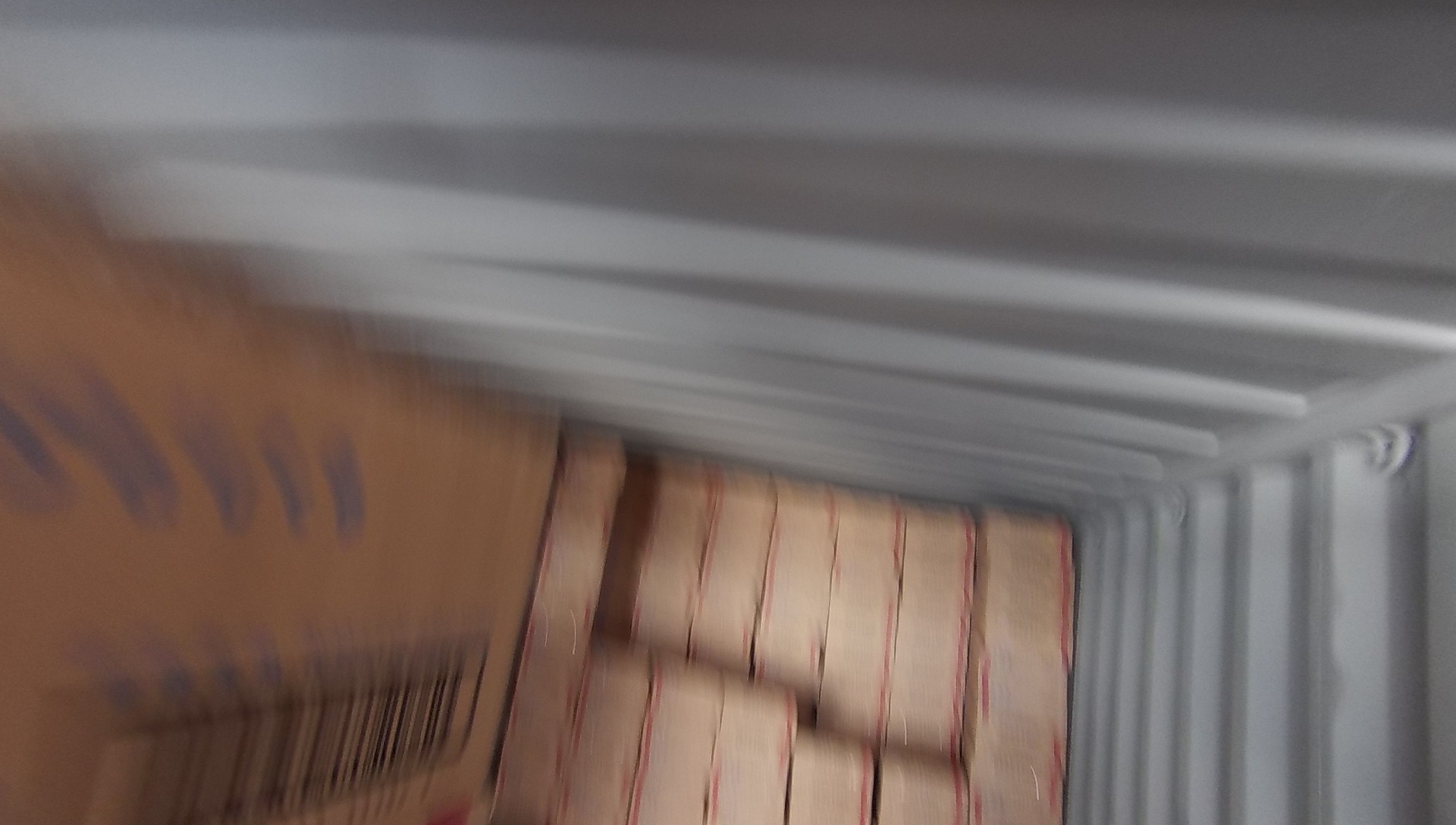The photograph features a notably blurry image that initially appears to capture a corner space, possibly a storage unit or a porch area. To the left-hand side of the image, there is a brown cardboard box prominently displayed, marked conspicuously with a large black barcode. Amidst the blur, some blue-font text is visible on the box, but it is too distorted to decipher the wording. The top and right side of the image show a corner where various gray, textured, striped surfaces intersect, hinting at structural elements that resemble the walls of a storage unit or the panels of a garage door. At the photograph's base, there is a discernible stack of light-colored stones or bricks, adding to the image's rough, utilitarian feel.